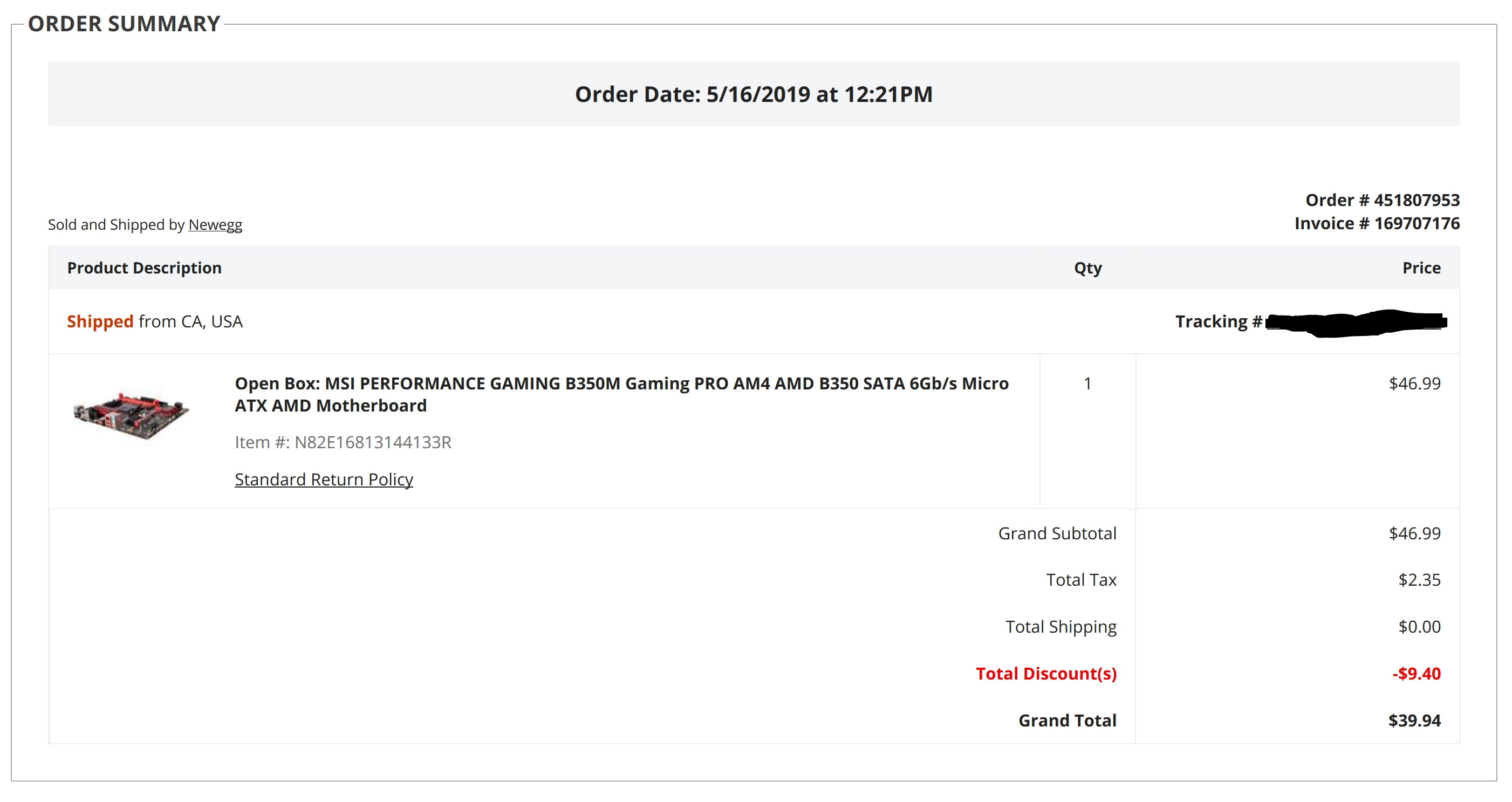This image features a detailed order summary from Newegg, captured on a white screen. The header at the top reads "ORDER SUMMARY" in prominent black capital letters, enclosed within a rectangular border. Inside the rectangle, there's a light gray horizontal strip that displays the order date "5/16/2019 at 12:21 PM" in black text. Below, it states "Sold and Shipped by Newegg."

The summary proceeds to list specific order details such as the "Order Number" and "Invoice Number" on the right side. The main body beneath these headings provides a breakdown, starting with product information. In red text, the status "Shipped from CA, USA" is indicated. Accompanied by a small graphic thumbnail, the item is described as an "Open Box MSI Performance Gaming 8350M Gaming Pro AM4 AMD 8350 SATA 6 GB Micro ATX AMD Motherboard." Further details include an item number and the mention of a "Standard Return Policy."

The order summary specifies a single unit purchased at a price of $46.99. Beneath this, a detailed cost breakdown reveals a grand subtotal of $46.99, a tax of $2.35, and free shipping. A discount of $9.40, highlighted in red, brings the final grand total to $39.94 in bold black text.

This meticulous order overview captures every aspect of the purchase, from the total cost down to shipping and discount details.